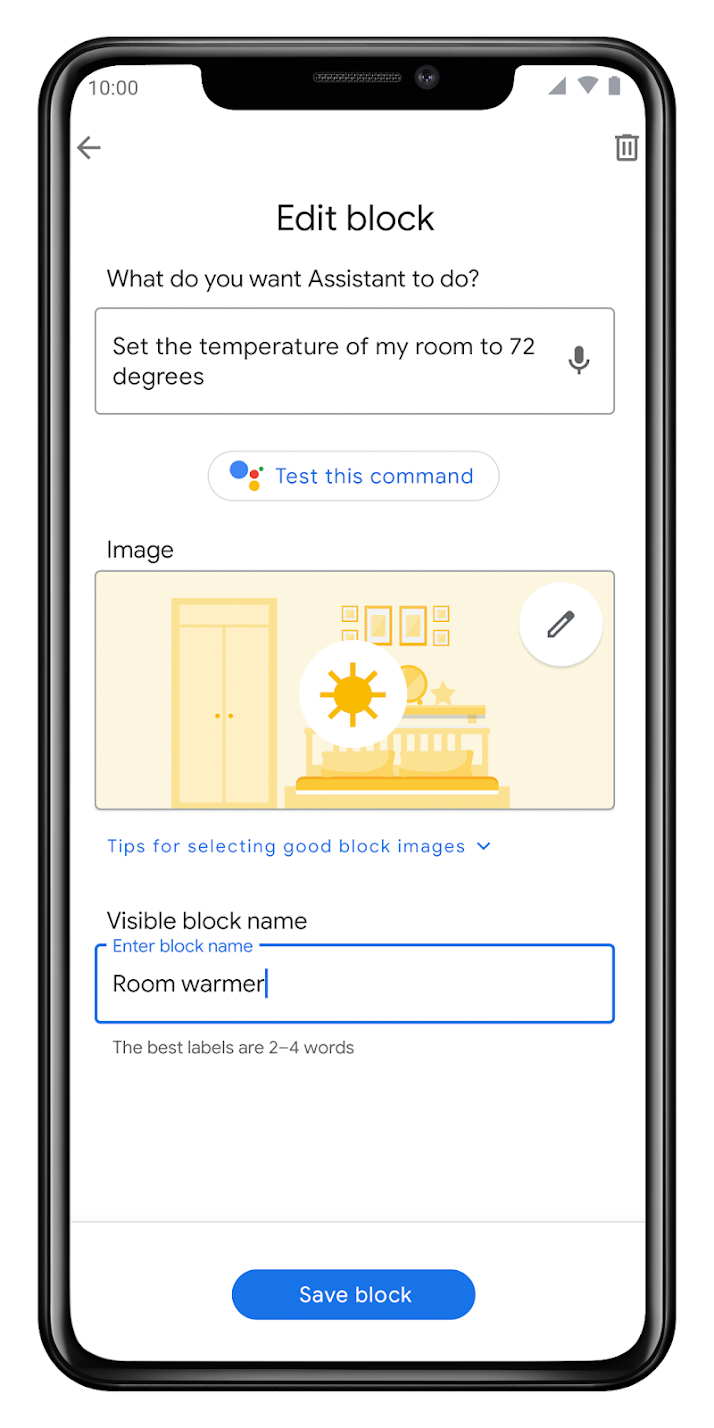The image features a smartphone screen displaying a user interface for a home automation app. In the upper left corner, the current time is shown as 10 o'clock. Next to it, there’s an arrow pointing to the left with the label "Edit Block." Below this, there is a prompt asking, "What do you want the assistant to do?" followed by a suggestion, "Set the temperature of my room to 72 degrees," and an icon of a microphone for voice commands.

Below this section, there's an invitation to "Test this command" accompanied by a blue circle. Adjacent to this, an "Image" icon reveals a small preview with a yellow door, a sun inside a circle, some pictures on a wall, and a bed. There's also a circle with a pencil inside, suggesting an edit option.

Further down, there's a section titled "Tips for selecting good block images" with a downward-pointing arrow. There’s a field labeled "Visible Block Name" for entering a name, and a search bar displaying the term "Room Warmer." Beneath this, there's a note recommending that the best labels are 2-4 words long. Finally, a blue circle containing the option to "Save Block" is located at the bottom.